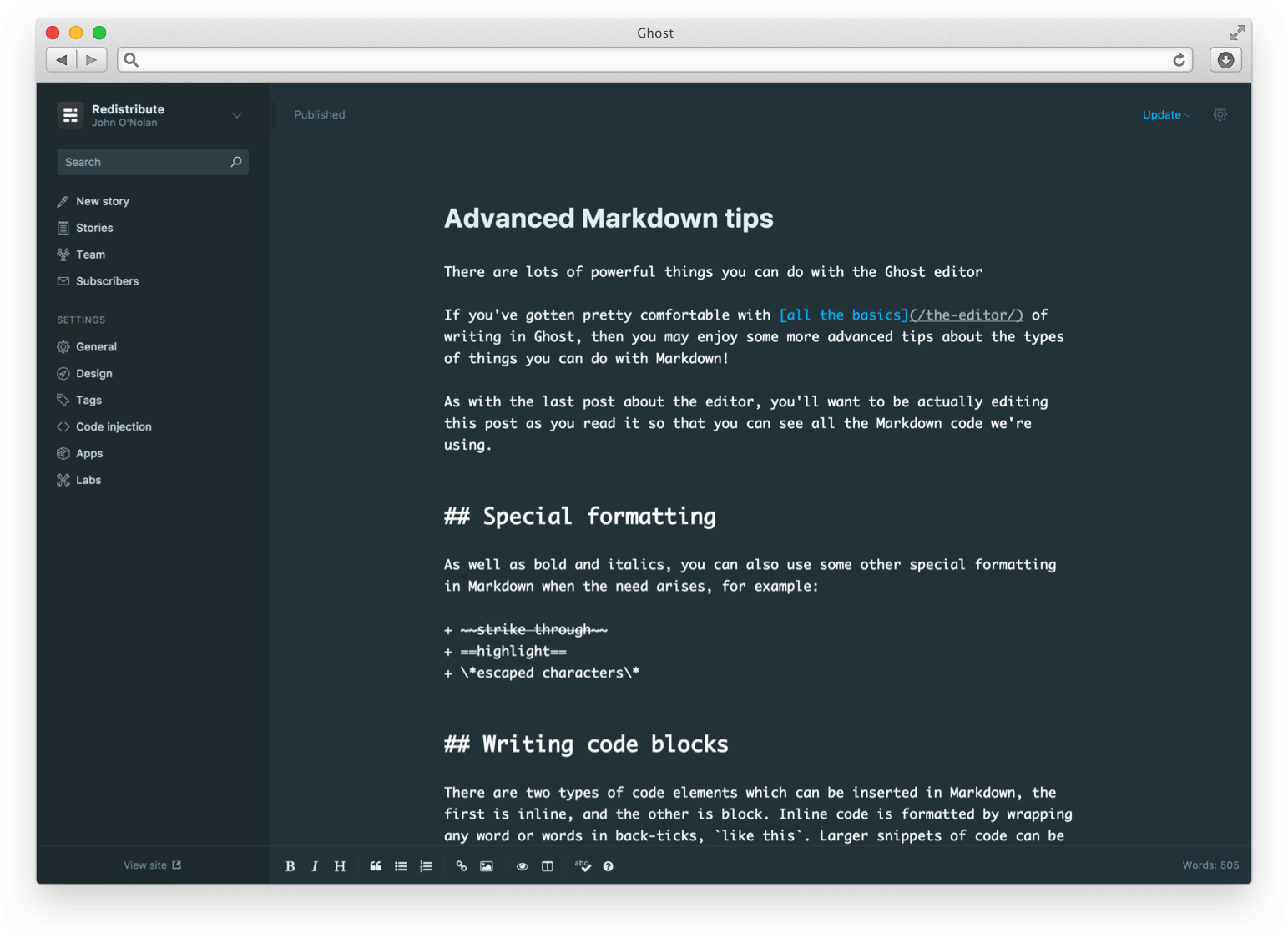This is a detailed screenshot taken from a desktop or laptop, specifically a Mac computer. The screenshot features a section of text titled "Advanced Markdown Tips." The text elaborates on the powerful functionalities available in the Ghost editor, aimed at users who are already comfortable with the basics and are seeking more advanced tips for writing in Markdown. 

The text encourages readers to actively edit the post as they read, providing hands-on learning for using Markdown code. It covers various special formatting options such as bold, italics, and strikethrough, as well as highlighting and escape characters. Additionally, the text mentions code formatting in Markdown, explaining that there are two types of code elements: inline and block. Inline code is formatted by wrapping words in backticks, while larger code snippets can be... The screenshot cuts off at this point, leaving the explanation of larger snippets incomplete.